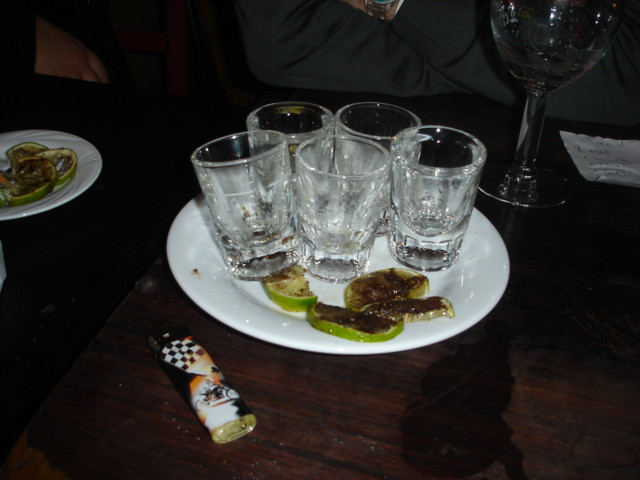In a dimly lit room, a photograph captures a richly textured scene centered on a dark wooden table. Dominating the composition, a small white plate holds five clear shot glasses, their surfaces streaked with residue, hinting at recent use. Nestled in front of the shot glasses are four slices of lime, their edges blackened, possibly from grilling, with one slice appearing slightly dirty. The plate and its contents rest atop the table, where a noticeable wet spot suggests a recent spill. In front of the plate, a distinct black and orange Bic lighter adorned with a race car flag design contrasts sharply with the table's dark wood.

To the left, a second, less prominent white plate is partially visible, holding only additional blackened lime slices. On the right side of the table, a partially filled wine glass contains a small amount of red wine, adding a splash of color to the dim scene. The background reveals a few people's arms, leaning casually against the table, hinting at a social atmosphere. Overall, the photograph's central focus remains on the white plate with the shot glasses and limes, set against the dark, textured background of the wooden table.